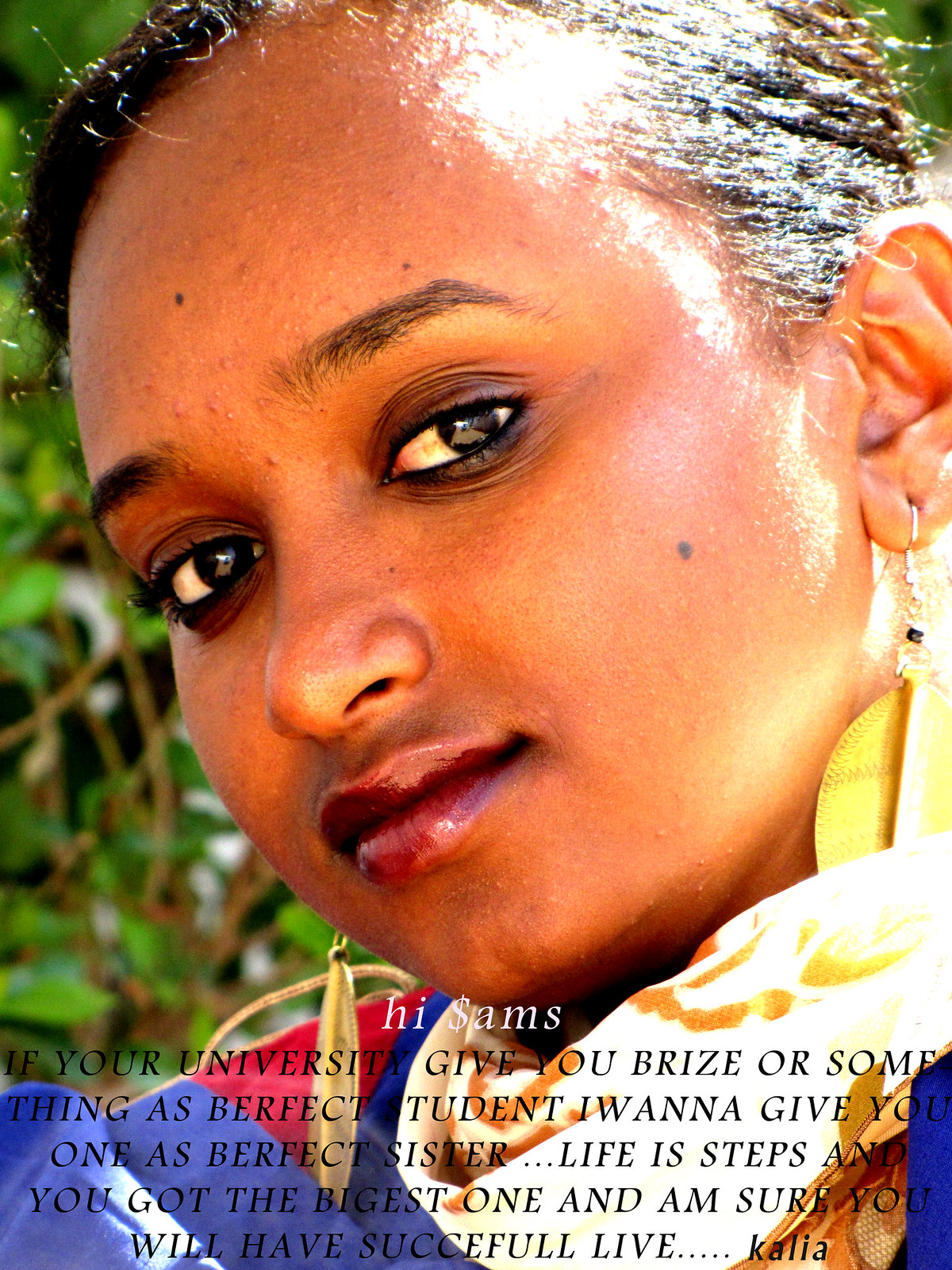The image features a young woman of Indian descent who is staring directly at the camera. Her dark brown eyes and brown hair complement her dark complexion. She is adorned with gold earrings, with one particularly notable in her left ear. She is dressed in a colorful robe or gown featuring hues of red, gold, white, and blue, along with a scarf. Her makeup includes eyeliner and lip gloss, adding to her vibrant appearance. Behind her is a backdrop of lush green vines, suggesting the photo was taken outdoors, with sunlight illuminating her. The bottom of the image has a heartfelt, albeit slightly broken, message in black text, reading: "Hi Sams, if your university gives you a prize or something as perfect student, I want to give you one as perfect sister. Life is steps and you got the biggest one, and I'm sure you will have a successful life. Kalia".